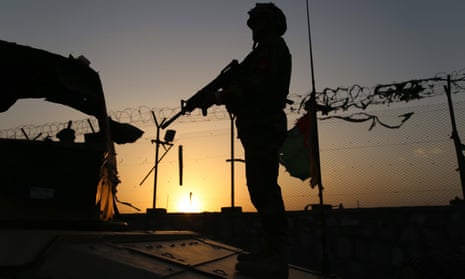The photograph captures the silhouette of a soldier set against the backdrop of a rising or setting sun, casting a dramatic gradient from bright yellow to dark blue. The soldier, standing tall and facing left, is equipped with a helmet and holds a gun pointed downward. Behind him, a high-security chain link fence topped with barbed wire extends across the scene, further emphasizing the austere setting. To the soldier's left, a small tented area with fabric sides is faintly visible. A tattered flag hangs from a flagpole near the fence, and scattered around the soldier are hints of military equipment, possibly a metal box and a vehicle, adding to the complex, shadowy landscape. The entire scene is bathed in the soft yet stark light of dawn or dusk, creating a powerful contrast that highlights the contours and features of the soldier and his surroundings.